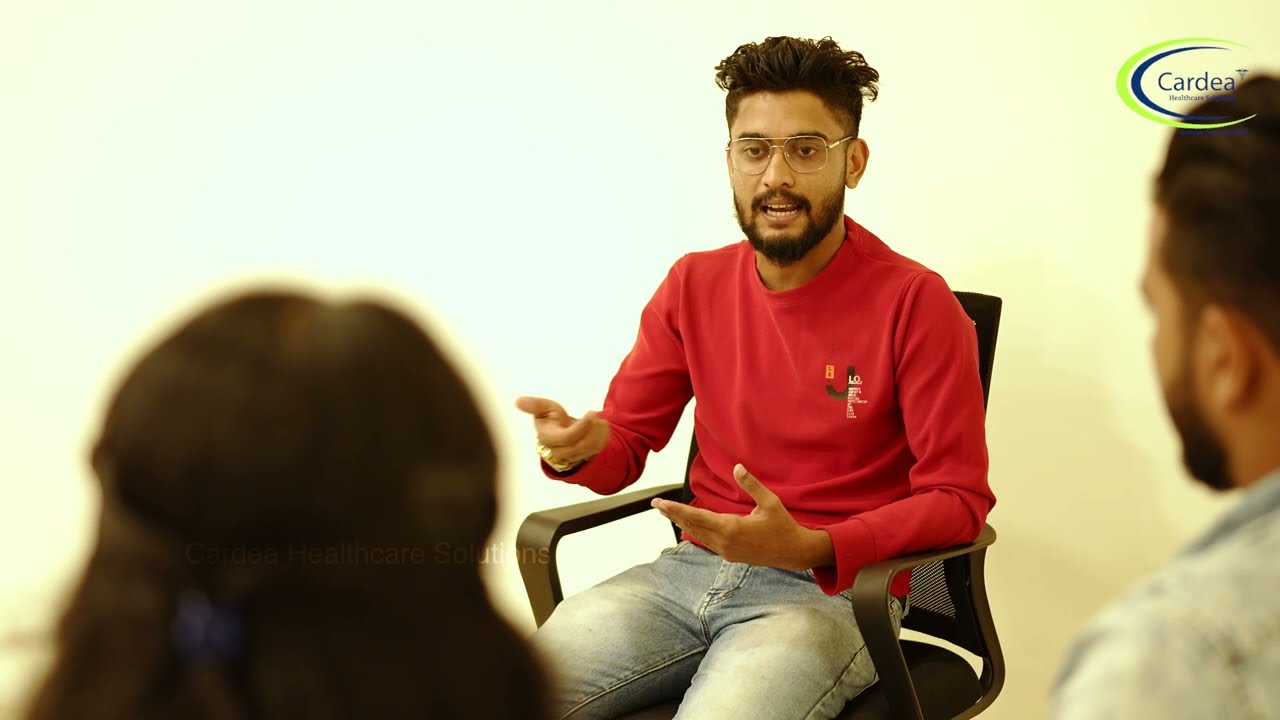In this image taken indoors, likely during the day in a work environment, three individuals are apparent. In the center, a South Asian man with caramel-colored skin, medium-length dark brown hair, and a brown beard sits in a black office chair with brown arms. He wears glasses with gold frames, a red long-sleeve shirt featuring a logo on the left side, and white-colored blue jeans. His body faces roughly the 7 o'clock position while his head is oriented towards the viewer, giving an impression that he is speaking or teaching. On the lower left, the back of a woman's head with long brown hair is visible. On the lower right, a slightly blurred man with short brown hair and a beard, mostly cut off from the frame, appears to be listening. He wears a white jean jacket and is oriented towards the 10 o'clock position. The color palette of the image includes white, brown, red, gold, light blue, and green. At the top right corner of the image, a logo reads "Cardia," encircled by a neon green incomplete oval with a blue half-moon shape on the left side of the word.